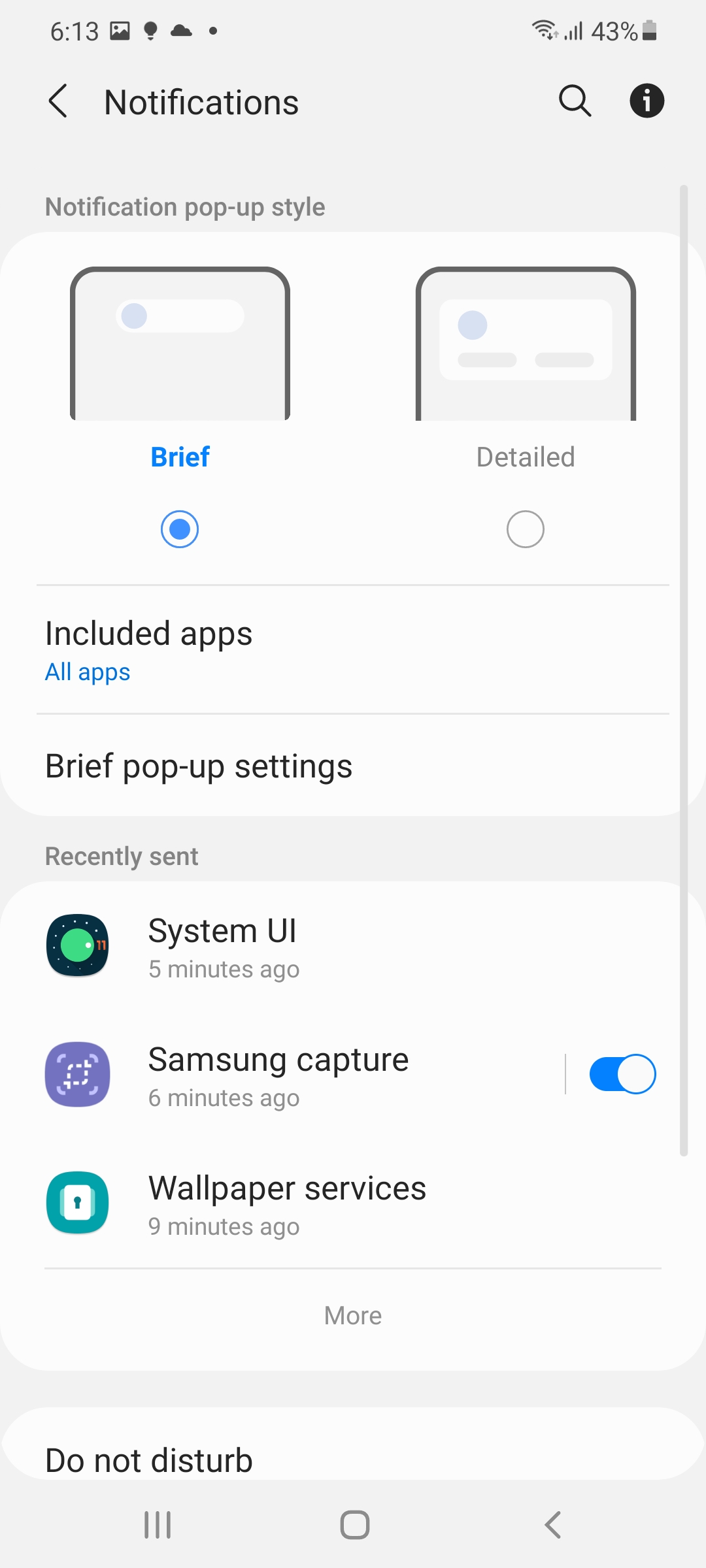The screenshot depicts a mobile phone, likely an Android device. At the top of the screen, the time reads 6:13. The status bar shows various icons: a photo, a light bulb, a cloud symbol, and a dot. On the right side, it indicates a Wi-Fi connection, cell service, and a battery level at 43%.

The displayed page is the notifications settings page. To the right, there are a search symbol and an eye icon, hinting at an info button. Below, the title "Notification pop-up style" is shown with two options: "Brief" and "Detail." The "Brief" option, which simplifies notifications into one bullet point, is selected and highlighted in blue. In contrast, the "Detail" option expands notifications into more points.

Further down, there's an "Included apps" section where "All apps" is highlighted in blue, suggesting that all apps follow the brief notification style. Beneath it, a "Brief pop-up settings" menu option is present but currently not displaying any content.

The "Recently sent" section lists recent notifications: "System UI" from 5 minutes ago, "Samsung capture" from 6 minutes ago (with a blue slider switched on), and "Wallpaper services" from 9 minutes ago. There's an option to click "More" to view additional recent app notifications.

At the bottom, partially visible, is the "Do not disturb" option. Also, the basic navigation menu is visible with the three-line menu button, a square, and a back arrow.